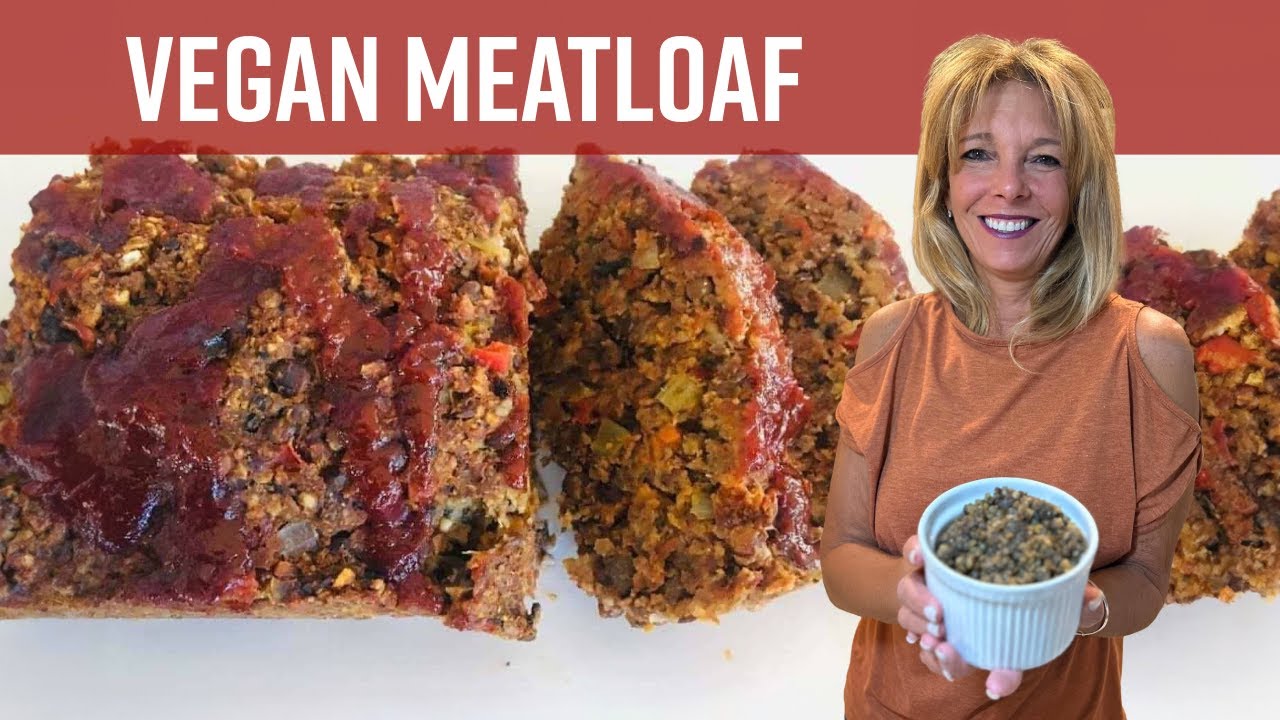This advertisement is set in a rectangular, landscape view with a vibrant red border. Dominating the top center of the image are the bold white words "Vegan Meatloaf." Below this text, there is a detailed photograph of the vegan meatloaf itself. The meatloaf, which is plant-based, displays a rich brown coloration and is interspersed with specks of orange, green, and black ingredients, suggesting a variety of vegetables. It is sliced into one large square piece followed by several smaller quarter pieces, all generously drizzled with a dark red sauce, resembling ketchup. 

To the right of this appetizing display, we see a cheerful woman, presumably the chef, who has shoulder-length blonde hair and is wearing a sleeveless orange blouse. She is holding a deep white bowl filled with the key vegetable ingredients of the meatloaf, suggesting freshness and home preparation. The woman is smiling warmly and looking directly at the camera, contributing a personal and inviting touch to the advertisement. The background surrounding the meatloaf image and the woman is a subtle mix of white and light gray, allowing the vibrant colors of the meatloaf and the chef's outfit to stand out.